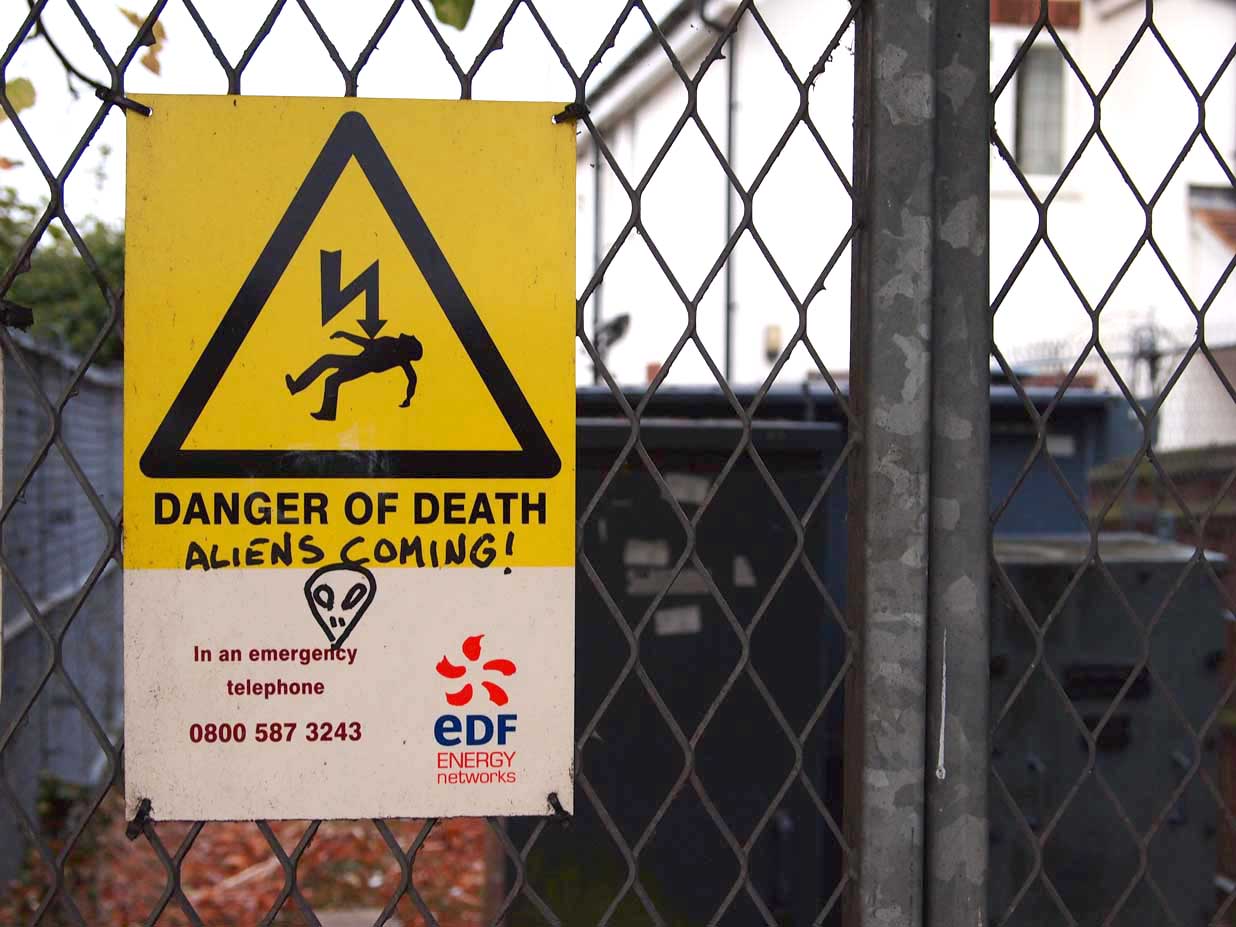The image depicts an outdoor setting with a steel chain-link fence held together by four zip ties. Attached to the fence is a prominently displayed warning sign that is divided into two sections: the upper three-fourths in yellow and the lower fourth in white. Central to the yellow area is a black triangle containing an image of a man being struck by an arrow, accompanied by the stark warning "Danger of Death." Below this, someone has used a marker to add graffiti, writing "Aliens coming!" along with a crude drawing of an alien face. The white portion of the sign contains red lettering that states, "In an emergency telephone 0800-587-3243." To the right side of this message, the letters "EDF" appear in blue, and below them, "Energy Networks" is written in red. Red splotches are visible above the EDF logo. The background reveals several metal boxes, a trash dumpster, a white house, and scattered leaves on the ground.